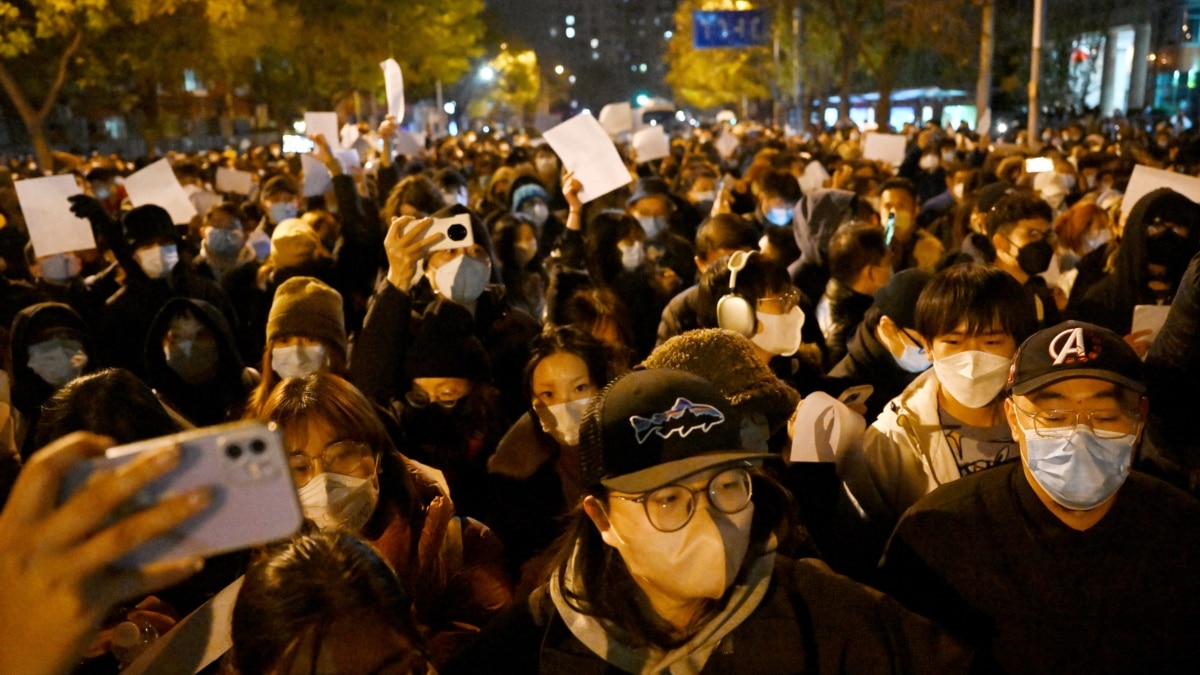In this nighttime city street scene, a large crowd of people, likely in an East Asian country such as Japan, China, South Korea, or Vietnam, stand facing forward, many holding up cell phones and white pieces of paper in the air. All are dressed in jackets and medical masks. Central to the image, a man wears a black hat adorned with a fish logo, round brown glasses, and a blonde mask. To his right, another man sports a black hat with an 'A', lighter silver square glasses, and a blue mask. Just behind, a man with dark black hair wears a white mask and coat. Further left, a woman with middle-parted brown hair dons a mask that's white on top and brown underneath. At the top of the image, in the back, a blue sign with the letter 'Y' and possible 'YWC' text is visible. Buildings and trees are faintly visible against the night sky, illuminated by city lights. The image is taken from a slightly elevated perspective, capturing the rows of masked individuals who are part of a probable protest. The colors in the image include black, beige, white, shades of blue, green, and greenish-yellow.